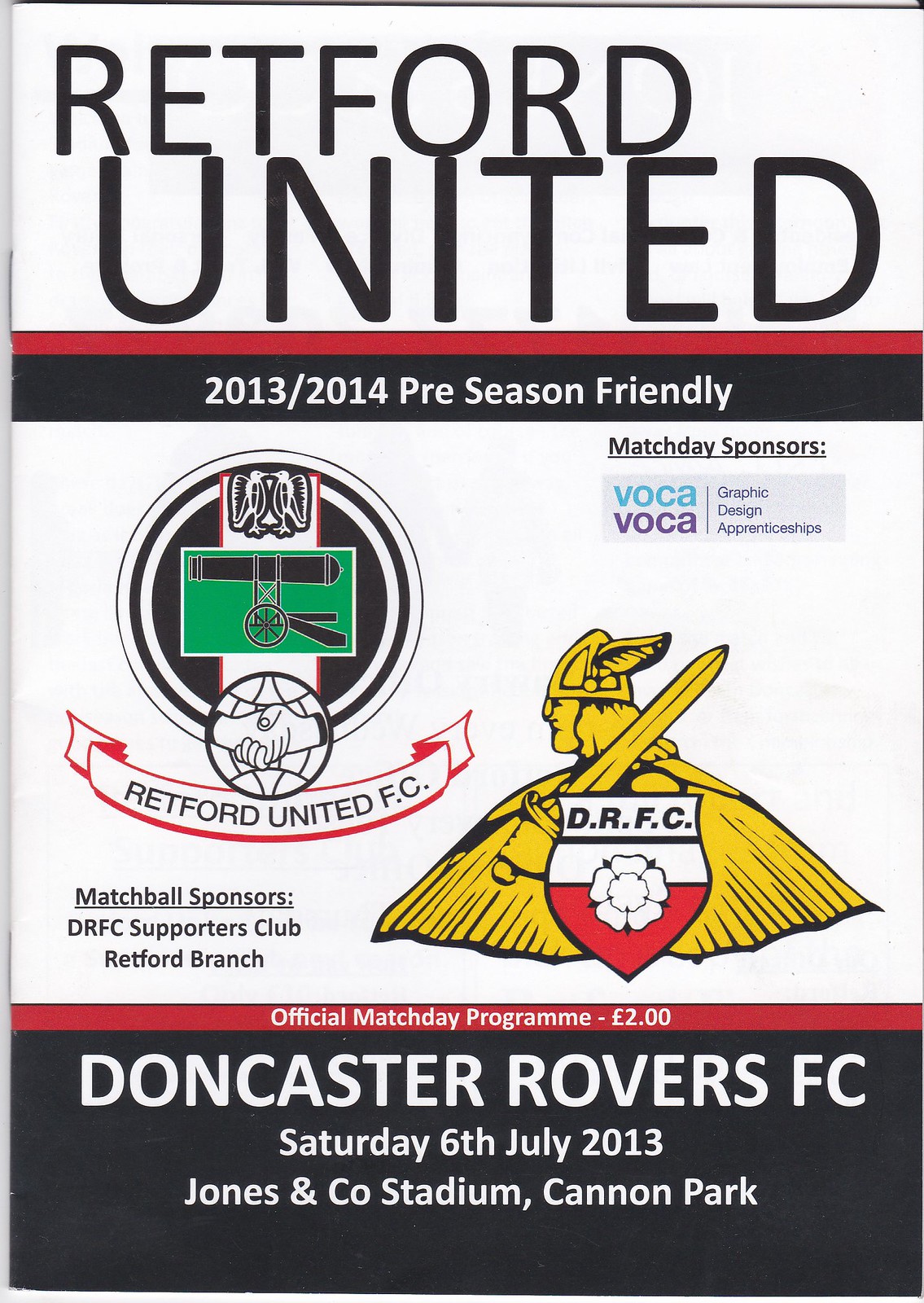This is a detailed poster advertising a preseason friendly event for Redford United FC. At the top, in bold black capital letters, it reads "Redford United." Below that, a narrow red line surmounts a black box containing the white text "2013-2014 Preseason Friendly." In the center, there are two prominent logos: on the left, a black circular emblem with various elements and the image of two hands shaking hands, symbolizing unity, and on the right, the DRFC logo featuring a helmeted figure wielding a sword and a shield on a yellow background. The poster lists "Match Day Sponsors: VOCA Graphic Design" and "Match Ball Sponsors: DRFC Supporters Club Redford Branch." Towards the bottom, another red line declares "Official Match Day Program, 2 pounds." The final section, presented on a black background with white text, provides event details: "Doncaster Rovers FC, Saturday, 6th July 2013," at "Jones & Co Stadium, Cannon Park." Predominantly featuring the colors white, black, and red, with touches of green, gold, and yellow, the poster effectively conveys all pertinent information against a white background with ample use of black text.